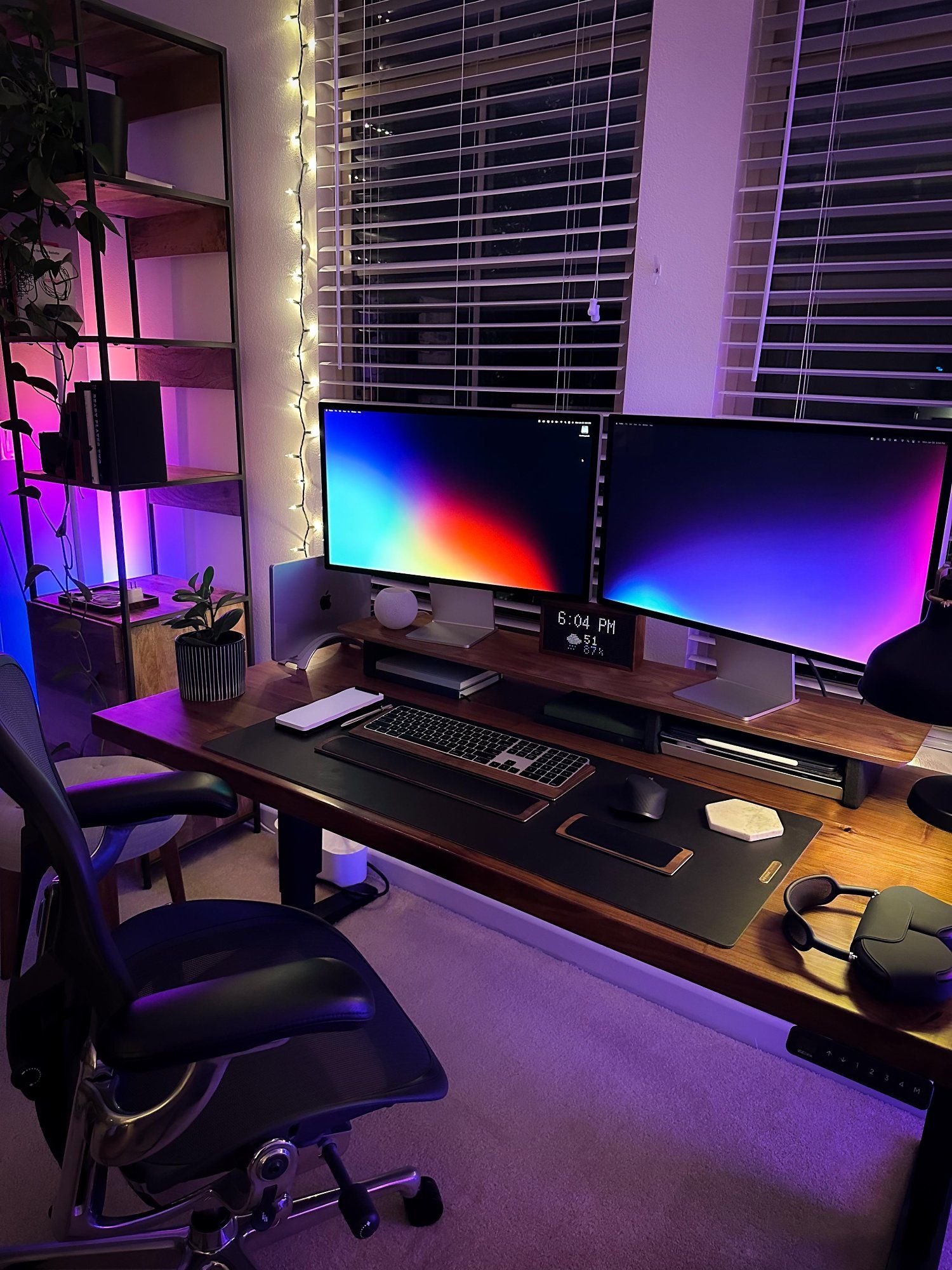The photograph captures a dimly-lit room, evoking a moody ambiance accentuated by various colored lights. Central to the image is a large, impeccably neat desk equipped with an ergonomic chair. Two substantial iMac monitors dominate the desk, their screens glowing with a vibrant array of colors—red, yellow, blue, and green on the left monitor, and purple, blue, green, and yellow on the right. The desk is organized with a keyboard, mouse, a pair of headphones, a phone, a small potted plant to the left, and possibly VR glasses or shades on the right. A pen and notepad lie near the plant, while a lamp with a lampshade sits nearby. Open Venetian blinds reveal darkened windows adorned with a string of fairy lights encircling them. In the corner stands a metal and wood shelf unit, hosting more plants and files, illuminated by muted pink and blue lights. The overall scene suggests a sophisticated and stylish computer setup, likely belonging to a gamer or a professional.